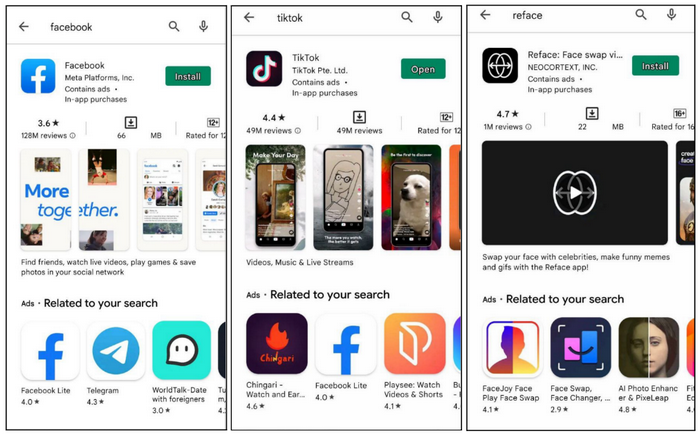The image depicts multiple screens of the Google Play Store on an Android smartphone. The first screen, positioned on the left, showcases the Facebook app with a prominent green "Install" button, indicating it is not yet downloaded on the device. The middle screen displays the TikTok app, featuring a green "Open" button, which signifies that the app is already installed on the phone. The third screen on the right highlights the Reface app, a face-swapping application, also accompanied by a green "Install" button.

Below these app listings, there are various promotional banners and advertisements for other applications, including Facebook, Telegram, WorldTalk, Chingari, PlaySee (for watching videos and shorts), FaceJoy, FacePlay, FaceSwap, FaceChanger, and AI Photo Enhancer. This layout is a typical representation of Google Play Store pages, where users can read app descriptions, see relevant promotional content, and either install or open apps depending on their current status on the device.